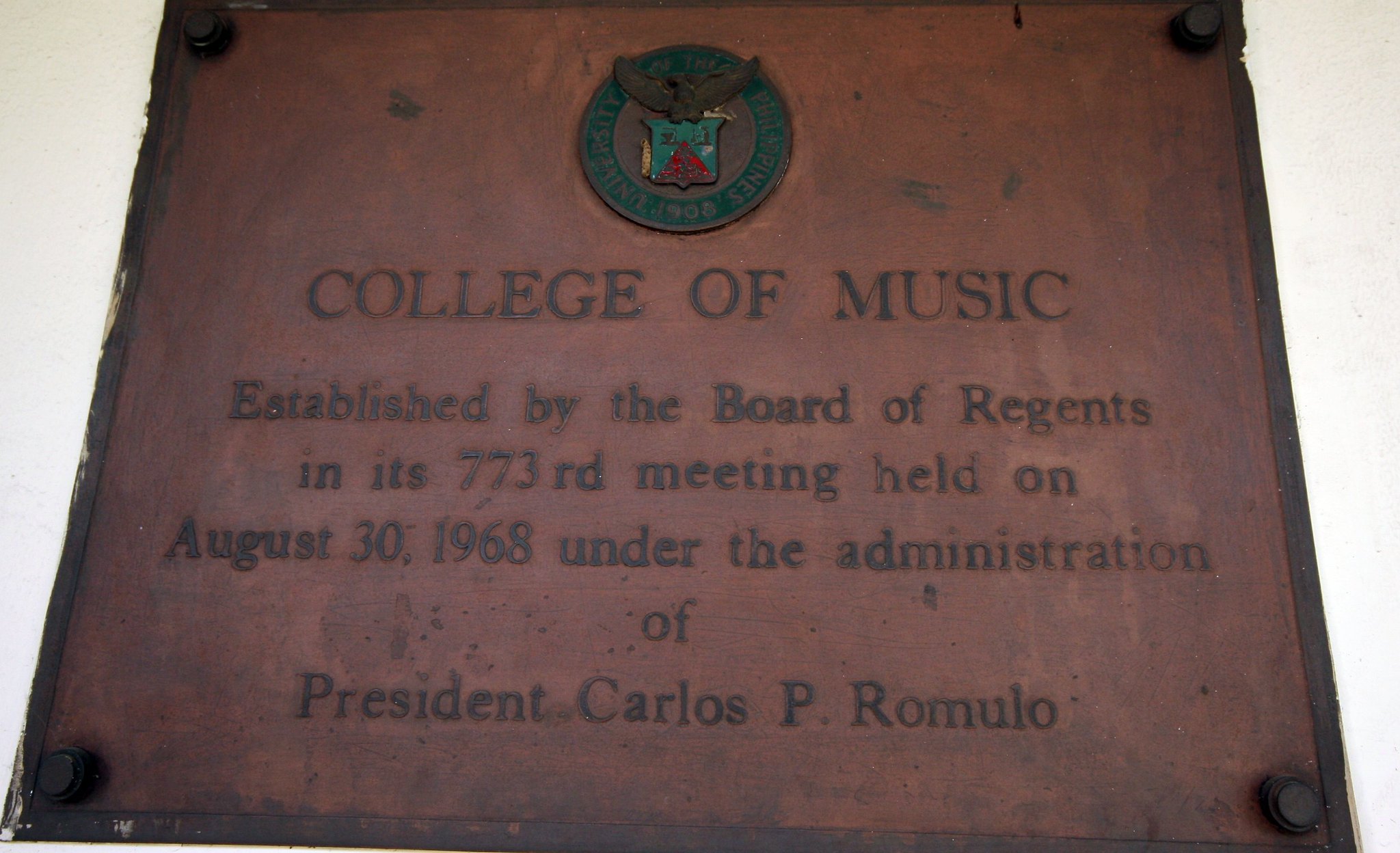The image features an antiquated plaque heavily weathered by time, evident from the conspicuous rust stains adorning its red surface. The plaque, fixed with four screws at each corner, exudes an air of historical significance. At its pinnacle, it showcases a round emblem depicting a dark-colored bird, likely an eagle, set against a turquoise backdrop. The emblem is intricate, containing undecipherable gray text and a shield divided into turquoise and red sections. The plaque reads: "College of Music, established by the Board of Regents in its 773rd meeting held on August 30th, 1968, under the administration of President Carlos P. Romulo." The detailed inscription and the emblem collectively narrate a tale of legacy and institutional pride.